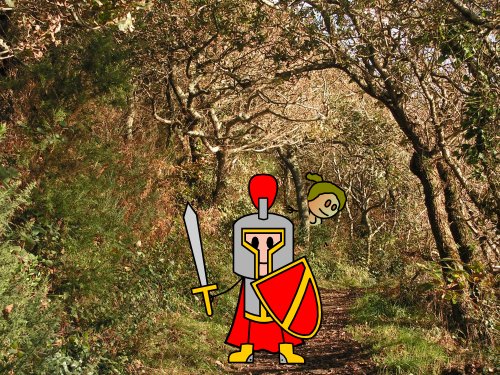In this artwork, a vibrant forest scene serves as the backdrop, showcasing a mix of green bushes and sparse, brown trees, creating a tangled, thorny appearance characteristic of fall. Superimposed on this realistic woodland setting is a cartoonish, stick-figure knight dressed in striking attire. The knight wears a red gown and cape, yellow boots, and a gray suit of armor accented with gold details. His head is adorned with a yellow helmet, topped with a prominent red feather. In his left hand, he holds a red shield featuring a bold yellow diagonal stripe, while his right hand grips a sword with a yellow handle and a gray blade. 

The knight's face, peeking out from under his helmet, has a pinkish hue and black eyes. Adding an intriguing layer to the scene, a mysterious female cartoon figure with greenish-bronze hair and strange pink eyes peeks out from behind the trees, a subtle smile on her face as she spies on the knight. This juxtaposition of detailed illustration against a realistic forest photograph creates a whimsical yet curious image, blending the boundaries between reality and fantasy.